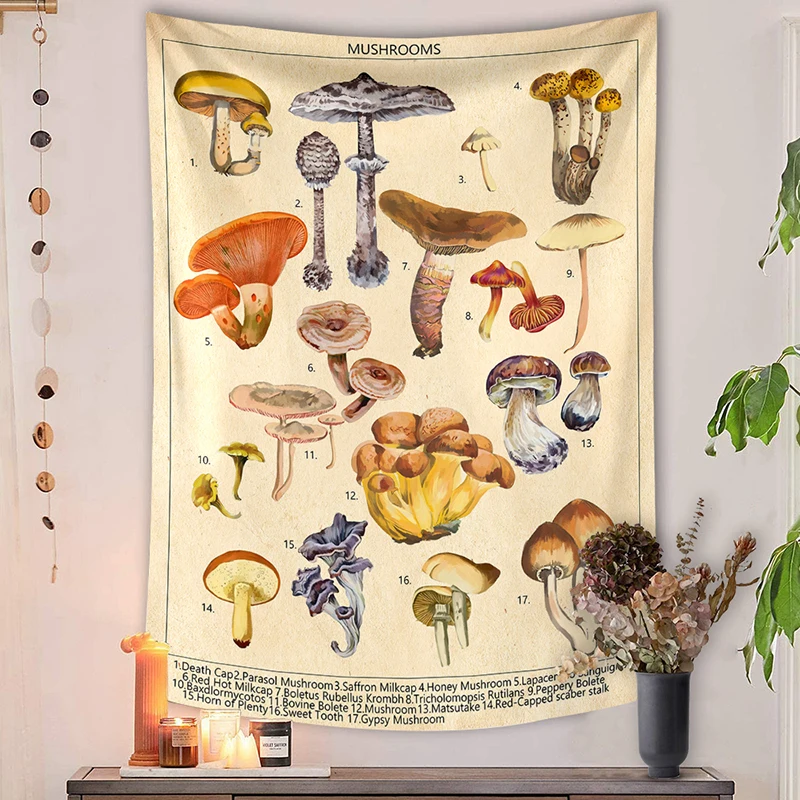The indoor photograph captures a neatly decorated white wall adorned with a square, light tan tapestry featuring an illustrated guide to mushrooms. The tapestry, framed centrally, bears the title "Mushrooms" in bold black print at the top. Below the title, 17 distinct, vibrantly colored mushrooms are depicted, each assigned a number from 1 to 17. At the very bottom, the tapestry provides a detailed key for identifying each mushroom. For instance, number 1 is the potentially deadly "Death Cap," while number 17 is the "Gypsy Mushroom."

At the bottom of the image, a sleek, long gray counter runs horizontally. The left end of the counter is decorated with a small setting of various lit candles. Adjacent to this setup, a string of shells hangs vertically from the wall, adding a rustic charm. On the right end, a decorative gray pot brimming with silk flowers sits beside a cascade of green plant leaves.

The detailed wall tapestry and its accompanying decor create a balanced, aesthetically pleasing composition. The mushrooms’ plethora of colors—ranging from red and orange to green and blue—along with their intricate details, provide a striking focal point, complemented by the ambient candlelight and natural elements on the counter.